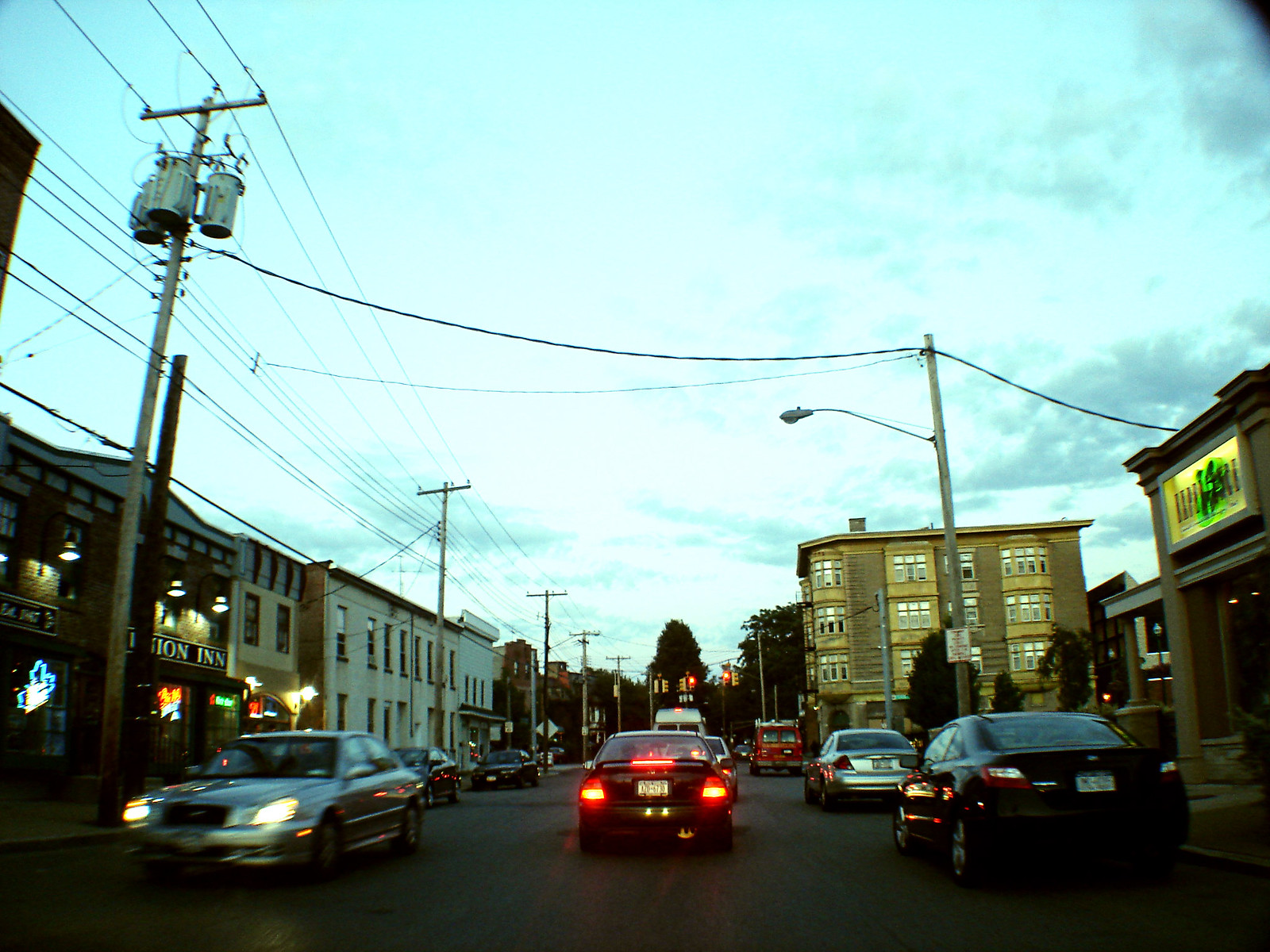This color photograph captures a bustling street in a moderately-sized town. The scene is vibrant, portraying a mix of old and new architectural styles. On the left side of the image, an older, quaint building stands out with a neon "Inn" sign above its door, suggesting it is likely a small hotel. The windows above the inn are illuminated with neon lights, adding a touch of warmth to the façade.

On the right side of the street, more modern buildings line the sidewalk, also adorned with neon signs above their entrances. The street itself is alive with activity, featuring several vehicles traveling in both directions. At the center of the street, a car is stopped, its taillights and brake lights glowing brightly, indicating a brief halt. Other vehicles are either parked along the sides or moving through the street, contributing to what appears to be a busy rush hour.

In the distance, a cluster of trees hints at a transition into a more residential area beyond the commercial hub. Above, the sky is mostly blue with a scattering of clouds, giving an overcast yet serene feel to the setting. Multiple utility poles with cables span across the street, emphasizing the functional aspect of the town’s infrastructure. Overall, the photograph vividly captures a moment of daily life in this active and diverse town.